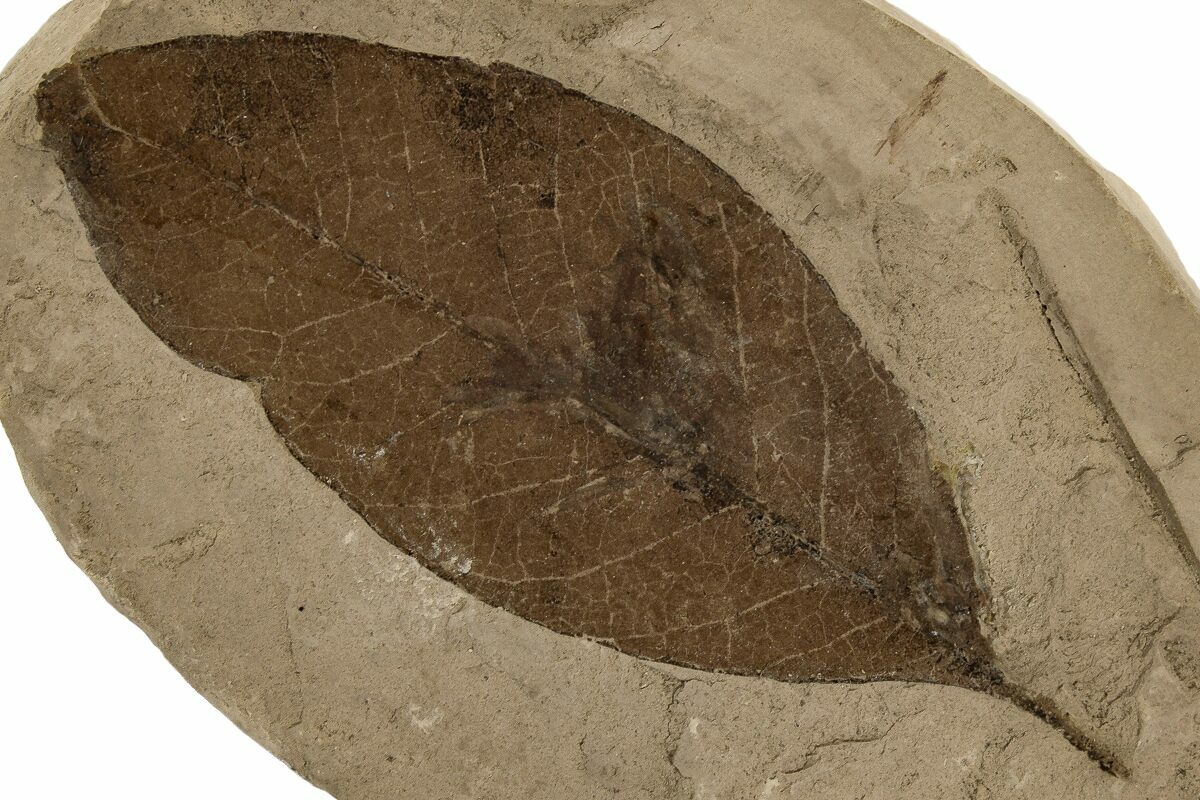The image captures a highly detailed, color photograph of a fossilized leaf embedded within a light brown stone, exhibiting a sepia tone. The leaf, positioned diagonally with its stem pointing to the bottom right corner, spans approximately two inches in length. Its dark brown color contrasts with the lighter, tan-colored stone that surrounds it. The leaf's veins are distinctly visible, and its surface is marked by areas of discoloration and darker smudges toward the middle. The stone itself exhibits an uneven texture with shades of black and darker brown scattered throughout. The overall appearance suggests the leaf might have been encased in concrete or a similar material, leading to its preserved, fossil-like state. No text or explanation accompanies the photo, leaving the origins and purpose of the image a mystery.